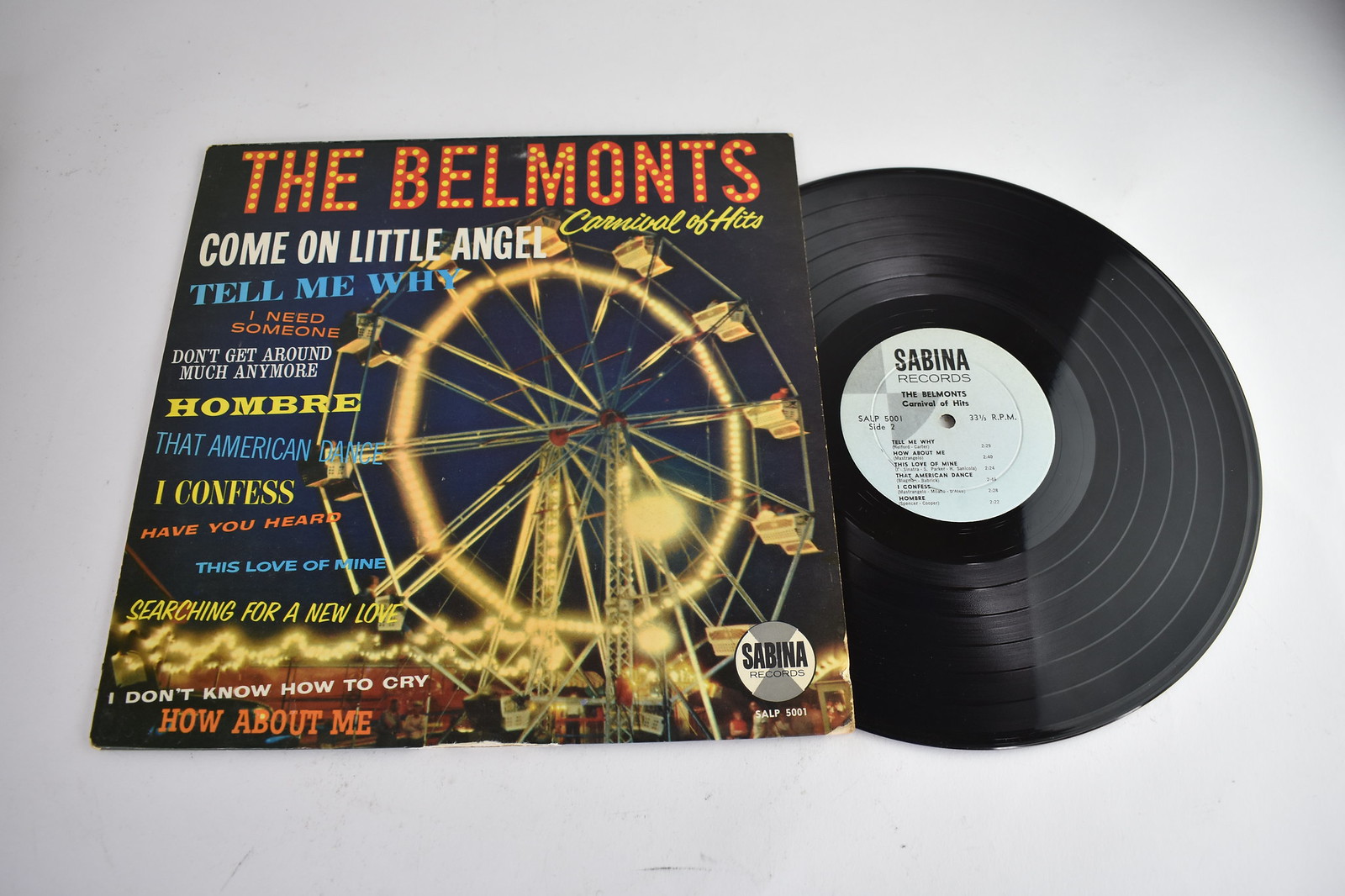In this indoor setting, possibly a record store, we see an image featuring a vinyl record and its cover laid against a solid gray background. At the center of the photo is the album cover of "Carnival of Hits" by The Belmonts, prominently displayed with a vibrant nighttime Ferris wheel and carnival scene in the middle. The album title and band name, "The Belmonts," are in bright, bold colors - white for the band name and a mix of orange, yellow, blue, and red for the track titles. The list of songs includes "Come On Little Angel," "Tell Me Why," "I Need Someone," "Don't Get Around Much Anymore," "Hombre," "That American Dance," "I Confess," "Have You Heard?," "This Love of Mine," "Searching for a New Love," "I Don't Know How to Cry," and "How About Me?" To the right of the album cover, the black vinyl record is visible, partially out of its sleeve, revealing a white center label that reads "Sabina Records" along with a track list. The overall composition, dominated by dark and bright contrasting colors, emphasizes the nostalgic essence of the physical record.